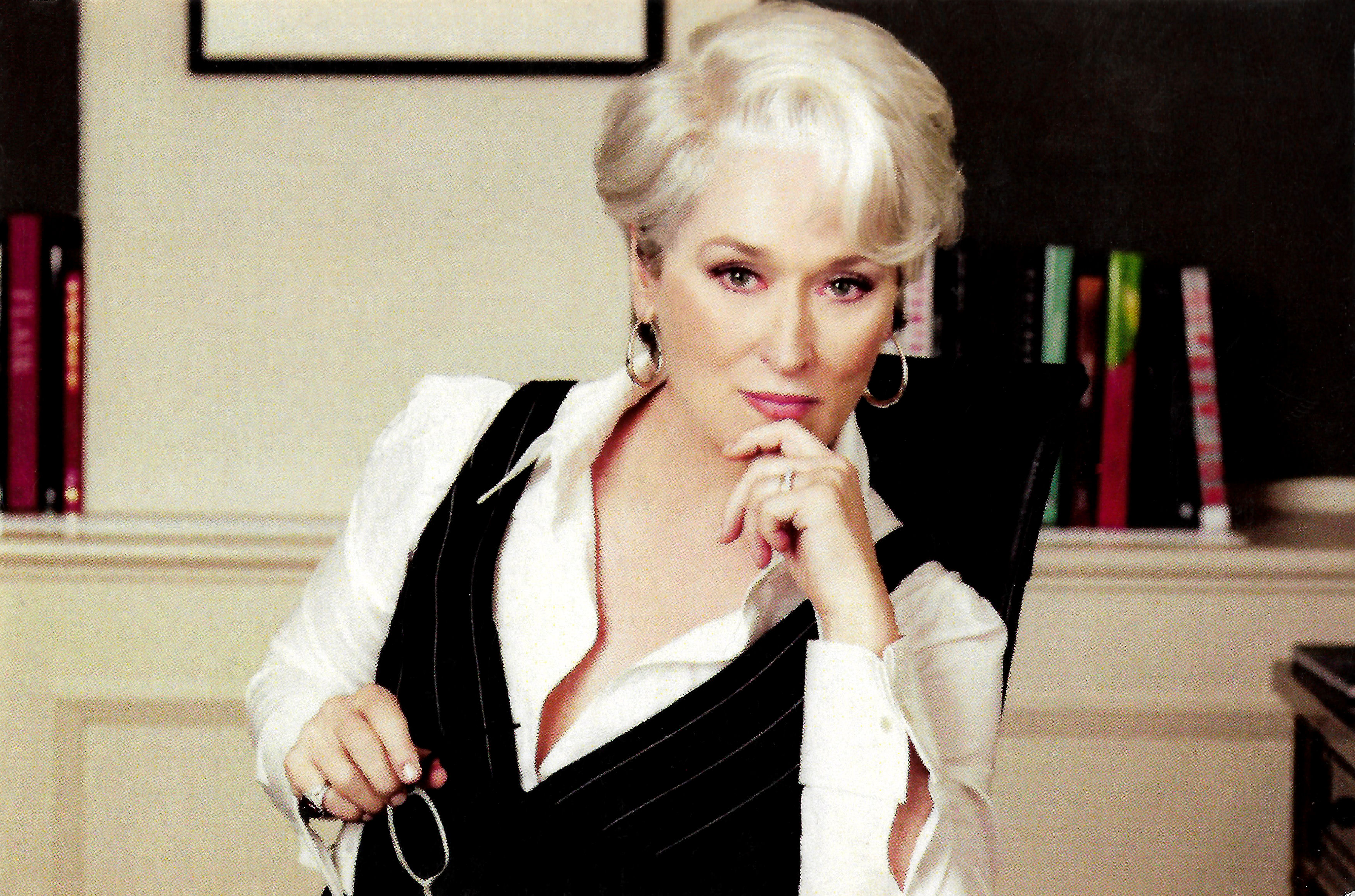This photograph captures Meryl Streep seated in a tall, elegant black chair with a high back, facing directly toward the camera. Her expression suggests deep contemplation as she holds a pair of glasses in one hand and touches her lips with the fingers of her other hand. Meryl's short, platinum blonde hair frames her face, revealing her large hooped earrings. She is dressed in a stylish ensemble featuring a white long-sleeve collared shirt, partially unbuttoned to reveal parts of her chest, and a dark, striped vest. The setting appears to be an office or a well-furnished room with off-white walls, white wainscoting, and visible shelving equipped with several books and a partially visible picture frame, all slightly out of focus in the background. Various colors, including black, white, and shades of tan, pink, red, green, and light blue, contribute to the composition of this seemingly vintage photograph.